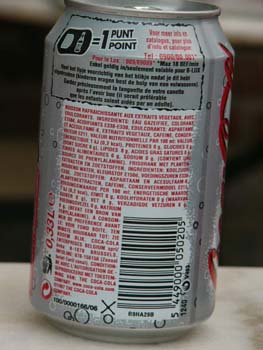This photograph is a super close-up and slightly blurry image of the back of a Coca-Cola soda can. The can itself is a steel gray color, with the iconic Coca-Cola logo in red that is somewhat visible on the extreme right edge. The photograph focuses on the back label displaying detailed product information and ingredients, which are mostly written in tiny red print on a large, white rectangle. The white rectangle is situated toward the bottom of the can and also contains a UPC barcode on the right-hand side, labeled 449000050205. In the upper part of the white box, there's a smaller white rectangle featuring some black outlines and both red and black text. Specifically, in one of the corners, it indicates that one of the pull tabs equals one punt point. The background of the image consists of a white table surface with some brown veining, and the upper part of the frame shows a dark brown background with a thin white strip across the top.